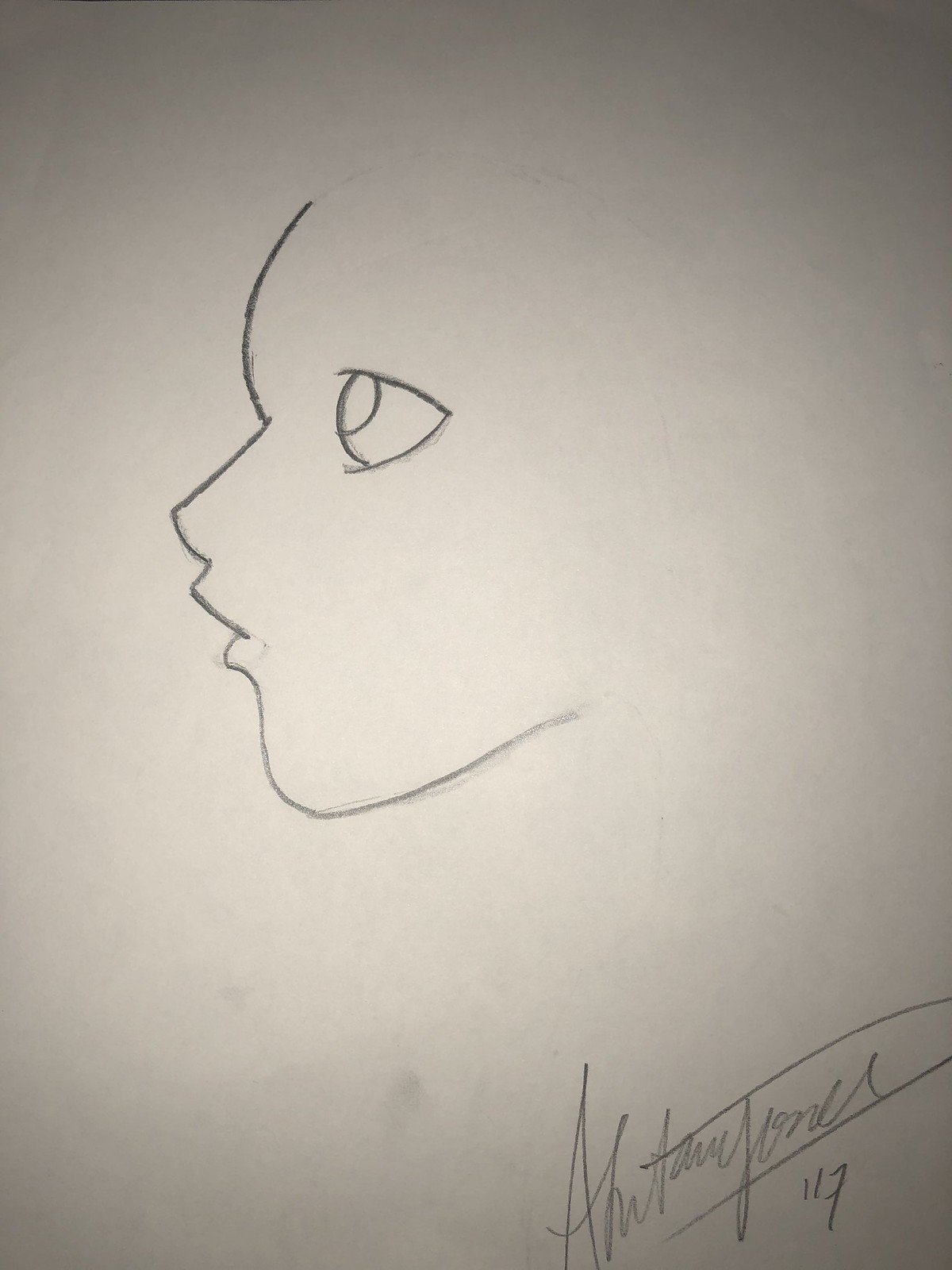The artwork features a minimalist, single-line drawing against a white paper background. Positioned in the bottom-right corner is a signature alongside the number "117." The portrait captures a face in profile, looking to the left, with the artist skillfully employing a single continuous line to outline the facial features. The line sweeps gracefully, forming the curve of the forehead, descending to outline the nose and moving inward to depict the lips before continuing down to sketch the chin and neck. The drawn eye gazes upward, imparting a sense of contemplation or curiosity. Adding depth to the simple yet evocative illustration, there are subtle, blotchy shadows beneath the chin and around the neck area. This delicate shading provides a nuanced sense of dimension and contrast to the otherwise straightforward line work.